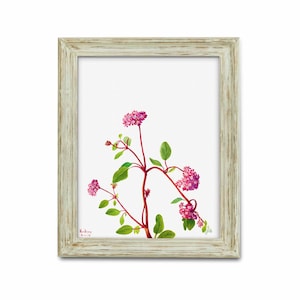The photograph features a small piece of framed wall art with a white, shabby chic distressed wooden frame, giving it a rugged and worn appearance. The artwork itself is centered within the frame and set against a plain white background. It depicts a delicate flowering plant that resembles a wildflower, showcasing a central stem adorned with multiple small, pretty pink flowers. The flowers are arranged with one prominently at the top, another bending slightly to the right, and a smaller one branching off to the left. The stem is a dark red hue, accented with several green leaves jutting out along its length. This charming and petite piece of art combines rustic charm and natural beauty, providing a simple yet elegant silhouette.